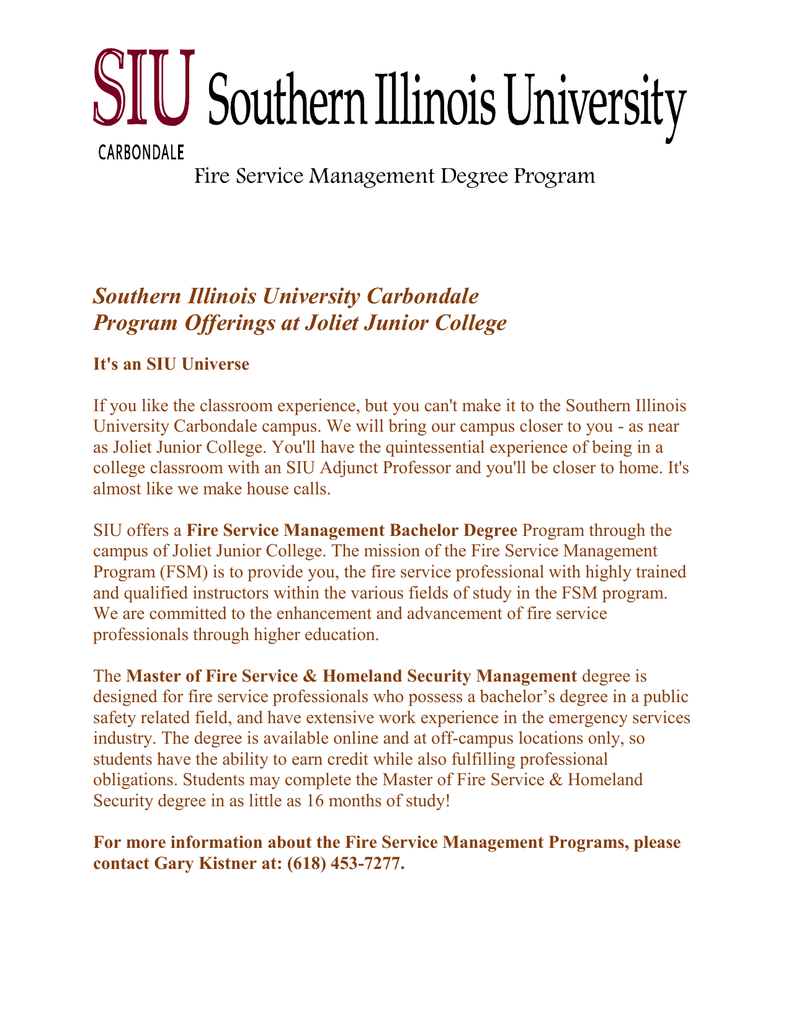**Descriptive Caption:**

Information Page for Southern Illinois University (SIU) Carbondale's Fire Service Management Degree Program.

This detailed information page on the Southern Illinois University (SIU) Carbondale website outlines the Fire Service Management Degree Program, focusing on its offerings at Joliet Junior College. The page emphasizes that SIU provides a versatile educational experience, allowing students to partake in classroom learning closer to home for those unable to attend the Carbondale campus. It highlights the availability of SIU adjunct professors who bring the authentic college classroom experience to Joliet Junior College, ensuring quality education is accessible locally. The program includes a Bachelor Degree in Fire Service Management and also delves into a Master of Fire Service and Homeland Security Management course. For further details or inquiries about the Fire Service Management Program, the page provides contact information, including a specific contact person and their phone number.